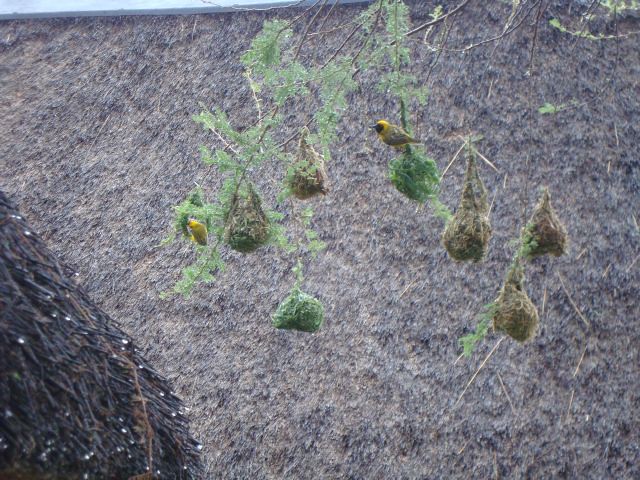This is a digital photograph featuring intricately woven bird nests hanging from a sparse tree branch extending from the upper left corner. The nests, some green and some brown, are roundish in shape and connected to the branch by elongated, triangular woven areas. A vibrant yellow bird with a black face and beak stands on top of one nest, while another bird of the same type is seen looking into another nest. The bird's plumage transitions into a greenish-gray body with a short tail. Surrounding this scene, the background is predominantly gray, with bits of dry, brown vegetation and prickly tree trunks visible in the lower left corner. Light green needles sparsely decorate the branch, adding a subtle hint of greenery to the otherwise neutral tones of the photograph.